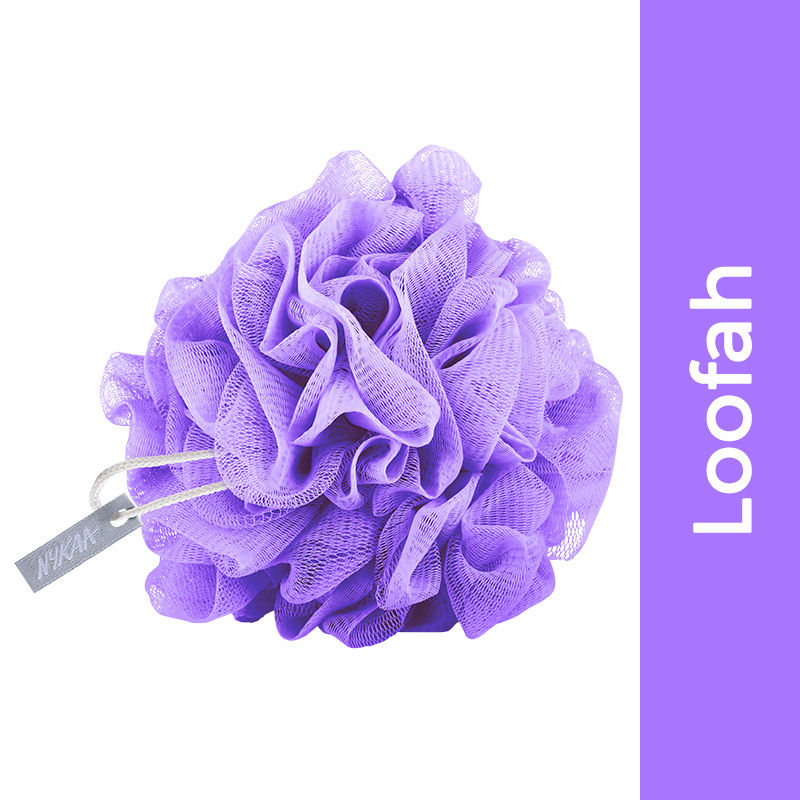The image features a detailed presentation of a purple loofah against a white background. The loofah, prominently positioned towards the left, showcases its intricately scrunched layers and weaves. Attached to the loofah is a small white nylon rope with a gray tag, which has the brand name NYKAA printed on it. Extending vertically along the right side of the image is a purple rectangular banner, with the text "loofah" in white, also oriented vertically. The overall composition is clean and minimalistic, focusing solely on the loofah and its branding elements, possibly intended for an advertisement or a product listing in a home and garden setting.